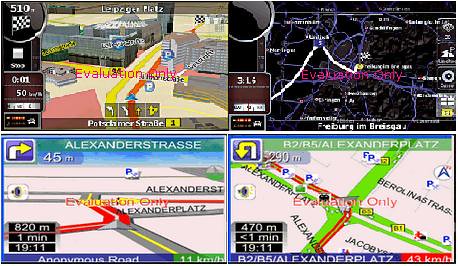The image displays a low-resolution computer screen divided into four equal rectangular sections, each showcasing a different navigation map. The top left section features a black map with yellow and red streets, building shapes, a parking sign, turn arrows, and some writing on the side. The top right section presents a black background map with bluish-purple roads and some different words. The bottom left section is a white map with green and red roads, showing the name "Anonymous Road" and mentions "Evacuation Alexander Strasse," alongside the numbers "820m" and "45M." The bottom right section also contains a white map with green and red roads, mentioning "B2/B5/Alexanderplatz" and "Berolinastrasse." Each map carries the label "evaluation only" on the front.